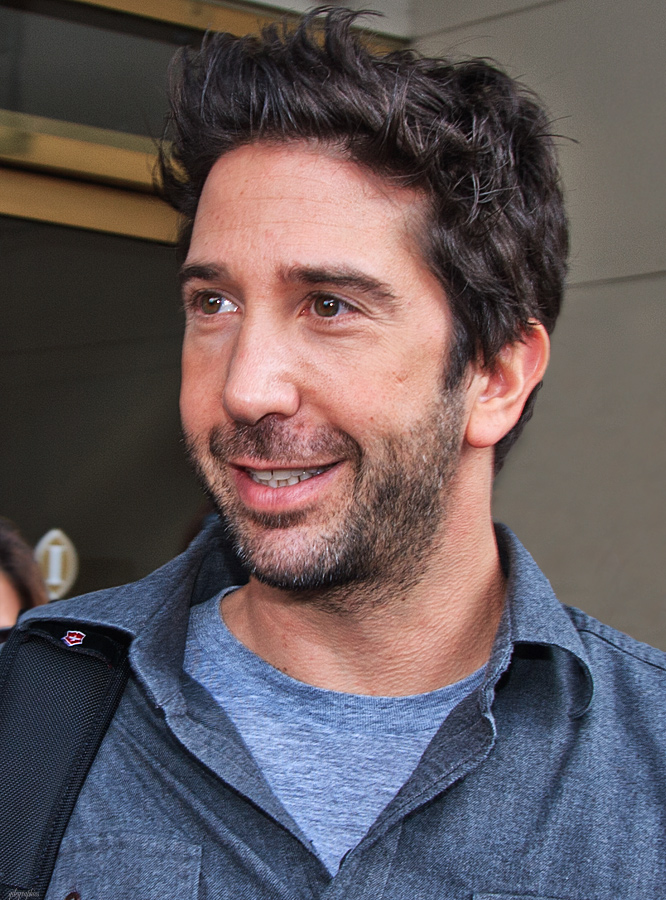The image depicts David Schwimmer, famous for his role as Ross in the 90s sitcom "Friends," standing centered in the frame. It is a recent, color photograph taken outside, possibly in front of the Intercontinental Hotel, as suggested by the emblem resembling an eye on the brown, brass-framed door behind him. The actor has medium-length, wavy, slightly unkempt black hair, and a scruffy beard and mustache indicative of several days' worth of stubble. Schwimmer is smiling and appears approachable, dressed casually in a blue jean button-up shirt over a gray t-shirt. He has a backpack slung over his shoulder featuring the Swiss Army logo, a red shield with a white cross. The composition hints at another person behind him, with only a glimpse of their forehead and brown hair visible. The photo is well-lit, possibly with flash, giving Schwimmer's face an even and smooth illumination.